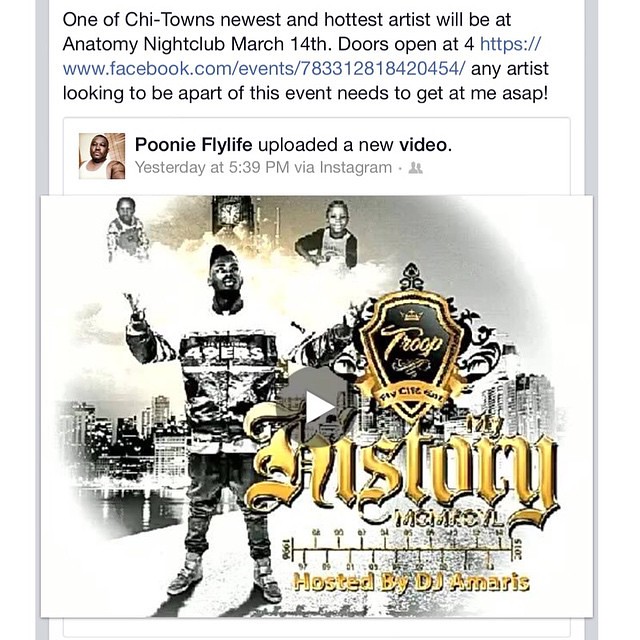The social media post, uploaded by Poonie Fly Life yesterday at 5:39 PM via Instagram, showcases one of Chi-Town's newest and hottest artists set to perform at Anatomy Nightclub on March 14th, with doors opening at 4 PM. The post features a detailed picture of an African-American man wearing a white feather, accompanied by a thumbnail image for a video depicting a black man in a 49ers jacket. Above the man, there is a grandfather clock and two children amongst clouds. The logo in the image looks like a shield and reads "Troop" with "History" in big gold letters underneath. The event is hosted by DJ Amorous, with text at the bottom reading "Hosted by DJ Amorous." For further event details, a Facebook link is provided: https://www.facebook.com/events/78331281842045. Any artists interested in participating are urged to contact immediately.